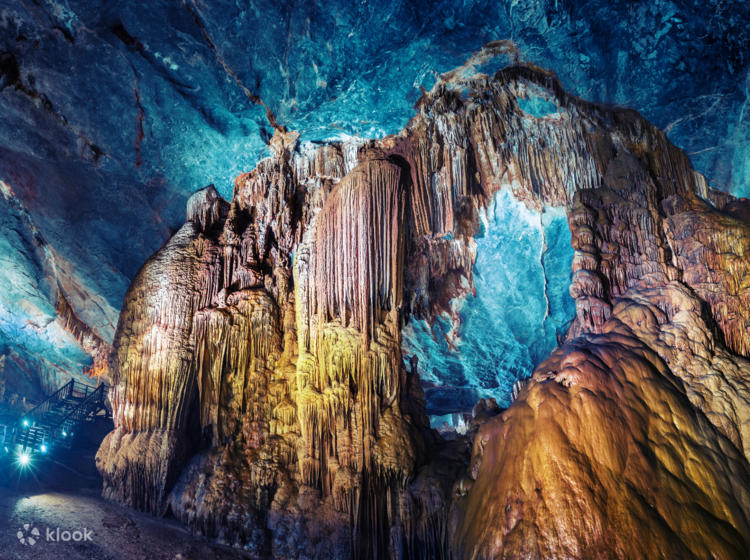This image depicts a majestic underground cavern with a blend of natural and artificial elements. Dominating the scene is a large, textured rock formation that angles outward and upward, with various colors such as blue, brown, beige, purple, and yellow. Some of these rocks have a sparkly blue hue, particularly in the background where another wall of rock is visible. The foreground rock is inscribed with the letters "K-L-O-O-K". The cavern's walls and ceilings are brightly lit in shades of blue, giving an almost ethereal atmosphere. At the center, there's a pool of water, adding to the mystical feel of the space. A small bridge or walkway, alongside a visible staircase, suggests that this is a place designed for tours. Man-made lights illuminate the scene, highlighting the natural beauty of the stalactites and arch formations with an orangish-yellow glow, transforming the interior into a surreal, fantasy-like landscape.